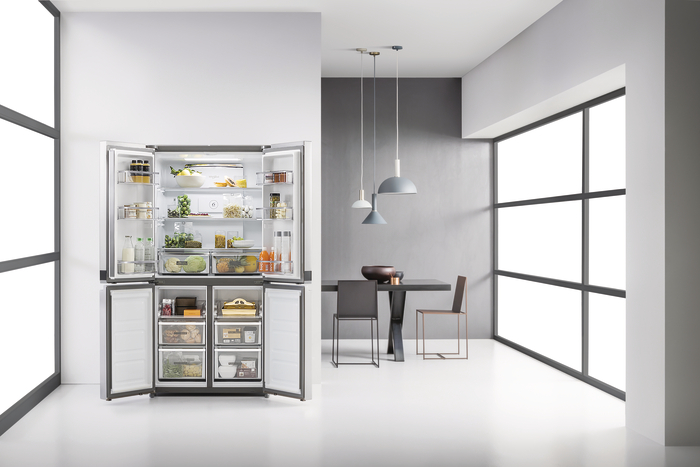This horizontal, rectangular image depicts an indoor room that resembles a converted garage turned into a hybrid office-living space. The walls are painted in varying shades of gray, transitioning from darker in the back to lighter at the front. Dominating the middle and right background is a table set with what looks like a typewriter, flanked by two chairs. Hanging above the table are three ceiling lights, each uniquely shaped: a larger circular light on the right, a triangular one in the middle, and a smaller circular light on the left, all in white. The room features prominent windows with black borders on both sides, enhancing the brightness of the space. A notable feature on the left side is a half wall, in front of which stands a cabinet filled with supplies. The cabinet has glass doors that are currently open, both at the top and bottom. While the details are slightly obscured by the image size, the refrigerator door standing ajar hints at its multi-functional use, blending elements of a kitchen, dining room, and office. The ceiling is white, complementing the room’s modern and functional design aesthetic.